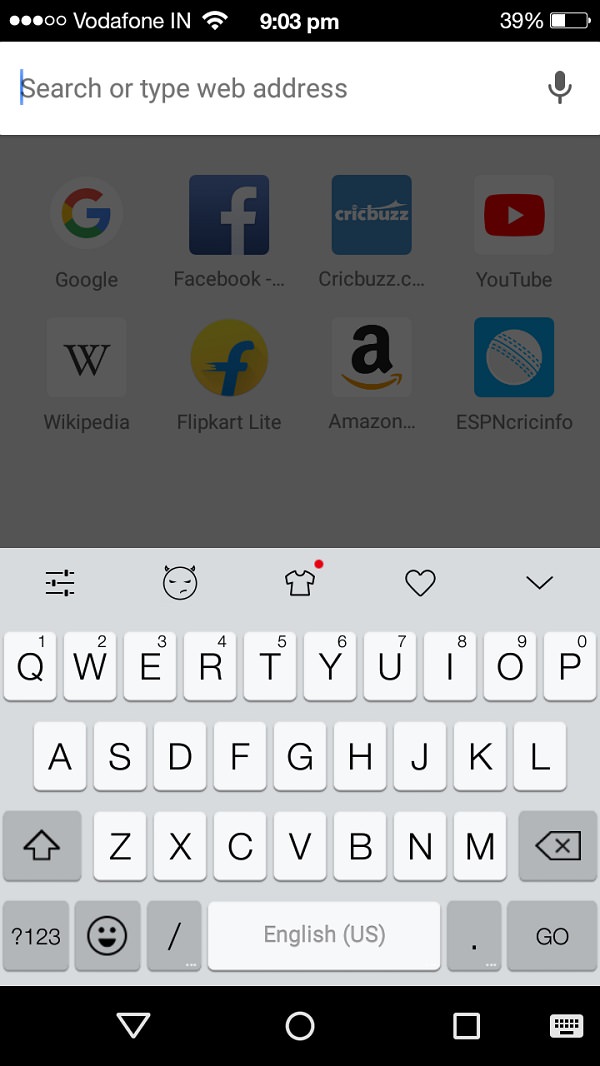Screenshot of a Vodafone phone in India, prepared for a web search at 9:03 p.m. with 39% battery remaining and three out of five signal bars represented by circles. 

The screen displays a browser page with a microphone icon on the right side of the search bar. The background is semi-transparent, showing a blurred view of various app icons including Google, Facebook, CrickBuzz, YouTube, SecondLine, Wikipedia, Flipkart Lite, Amazon, and ESPN Cricinfo, denoting a strong Indian presence with multiple cricket-related apps.

An overlay of a QWERTY keyboard occupies the lower half of the screen. The keyboard itself has a light gray background with white keys, featuring slight drop shadows for a 3D effect. Above the keyboard, several icons are visible, including a devil face, a T-shirt, and a heart.

At the very bottom of the screen, there is an emoji button next to standard navigation buttons: a down triangle, circle, and square, along with a keyboard icon on the far right. Additionally, the top icons are slightly obscured by a 50% black overlay, making them semi-transparent and blending into the background.